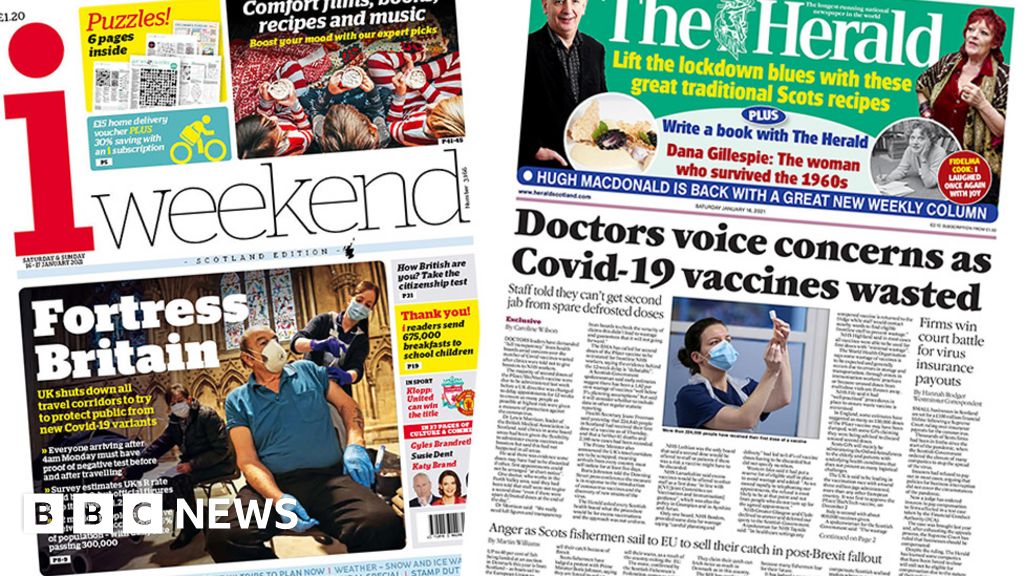The image features the front pages of two publications side-by-side. The one on the left is titled "i Weekend" and is identified as the Scotland edition. At the top left corner, there's a yellow section promoting six pages of puzzles, showcasing various types such as crosswords and word searches. Just below the title "i Weekend," there's a headline involving COVID-19. It reads: "Fortress Britain – UK shuts down all travel corridors to try to protect public from new COVID variants," with "BBC News" noted beneath it. Accompanying this headline is a photograph of a nurse administering a vaccine injection to a seated individual, with other masked individuals in the background. The setting appears to be a church, characterized by stained glass windows and ornate walls. On the right half of this front page, there is a preview of a feature promoting comfort foods, recipes, and music to boost moods, illustrated with an image of people in red and white striped pajamas.

The right-side paper is titled "The Herald" in white letters. Below the title, there's a section in yellow with the headline, "Lift the lockdown blues with these great traditional Scots recipes," accompanied by a picture of a white man on the left and a white woman with red hair on the right. Further down the front page, a prominent headline in large black letters states: "Doctors voice concerns as COVID-19 vaccines wasted." The main article is longer and includes a centered photograph of a nurse in a blue shirt and mask, holding and preparing a vial with a syringe.